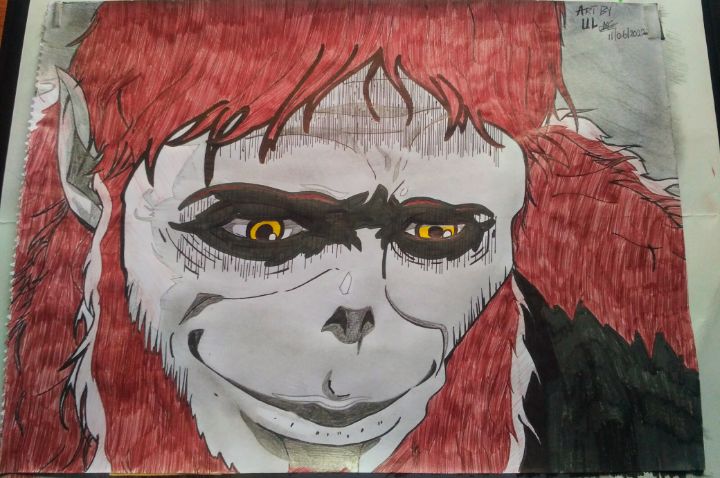The image showcases a hand-drawn, marker-colored poster featuring a unique creature that blends characteristics of an ape and a mythical being. The creature has long, flowing red hair that drapes down the sides and top of its head, accompanied by a matching red beard. The face, resembling that of a monkey or gorilla, has a prominent pair of pointy ears, much like those of an elf, with the right ear being particularly noticeable. Surrounding its yellow eyes with black pupils are distinctive black markings that extend around the eyes and across the bridge of the nose, giving the character a somewhat somber expression. The skin of the creature is light green, adding to its fantastical appearance. The creature's mouth is closed and has a pronounced size. The background of the drawing is white with black borders in the top left and right corners, and there is some jagged edging, reminiscent of a bubblegum wrapper, on the left side of the image. The upper right corner of the drawing features some illegible text.